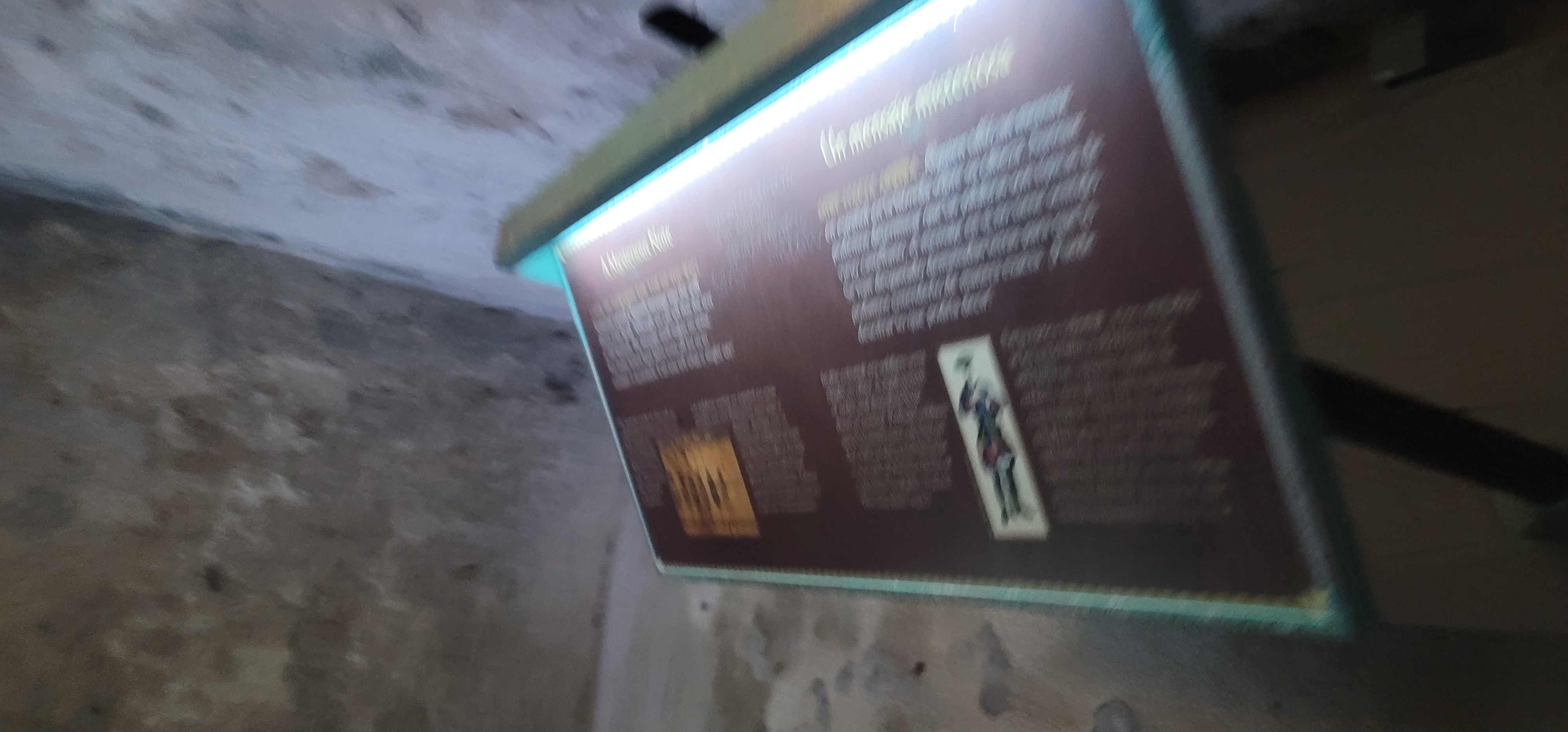A heavily blurred photograph capturing a desolate scene with rough concrete surfaces and noticeable signs of deterioration. The concrete walls and floor, marred with deep pockets and discoloration, display varied patches ranging from lighter shades to nearly black, possibly indicating water damage. Dominating the center of the image is a large, brown object, seemingly illuminated by a strip light. The object features white and yellow fonts, although the blur renders the text indecipherable. The object also displays some images: a dark, human-like figure set against a white background and an adjacent tanny orange image.